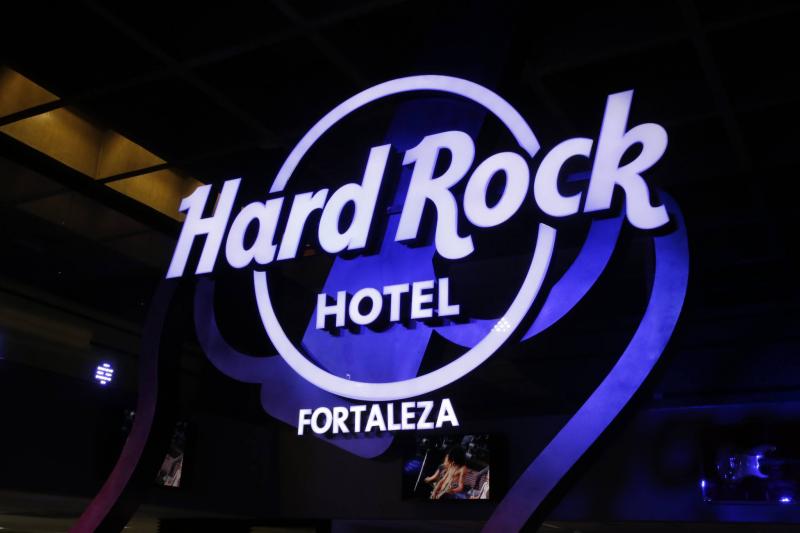The image showcases a sign for the Hard Rock Hotel at their Fortaleza location. The center of the image prominently features the iconic "Hard Rock" logo in its large, stylized font, with "Hotel" and "Fortaleza" written below it in white. The background is predominantly black, creating a stark contrast that makes the sign stand out. Surrounding the logo is a circle, within which lies a gradient outline of a Stratocaster guitar neck and body, shaded in hues of blue and purple, giving a dynamic, swirling effect. This deep purple and blue detail loops around the "R" in "Hard Rock" and extends to the left. The image appears to capture an indoor setting, with dim ceiling lights visible to the left and a shadowed guitar display to the right, accented by purple and light purple highlights. A screen showing an image is also faintly visible in the background, adding depth to the scene.